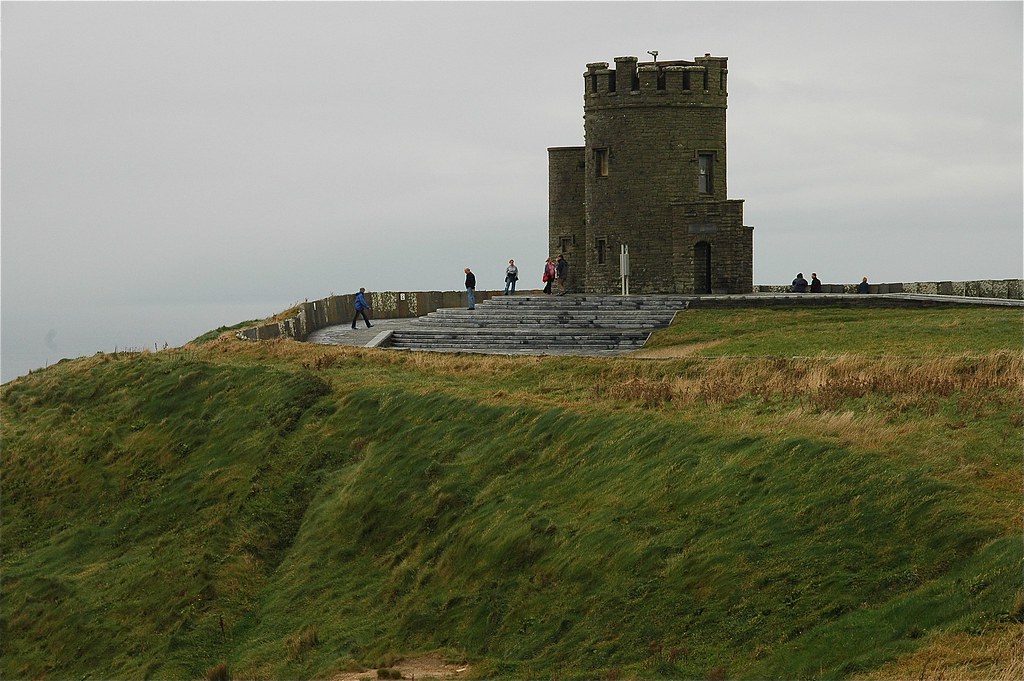This color photo captures a five-story, stone fortress situated atop a grassy hill, enveloped by a gray, cloud-covered sky. The ancient structure, possibly a lookout point, features a large staircase with around 20 steps leading up to its entrance, hinting at its historical significance. A wall encircles the fortress, and tourists can be seen exploring the premises. The backdrop suggests a distant body of water, possibly placing this fortress in a European country or the British Isles.